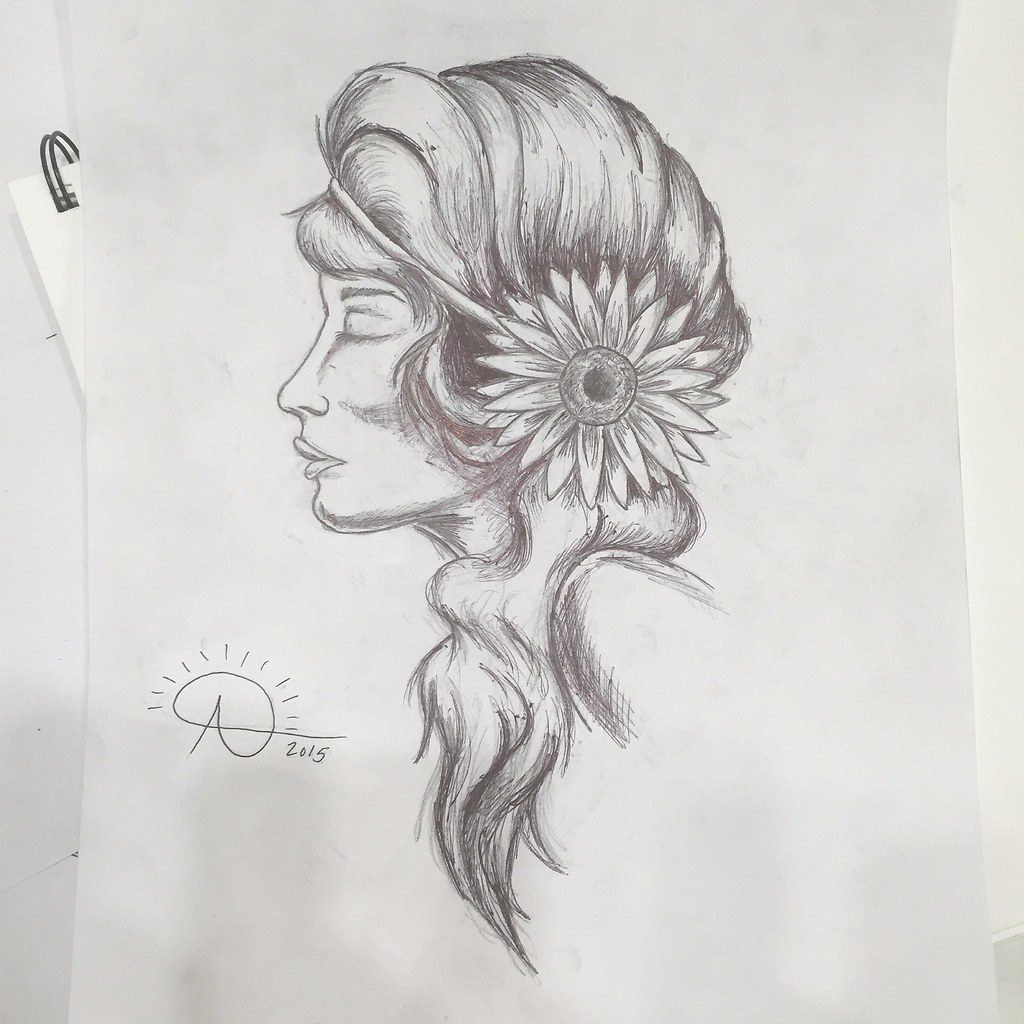A meticulously detailed black and white pencil drawing is showcased on a piece of paper at the center of the image. In the background, a notebook with black spiral binding is subtly visible. The artwork features a side profile of a woman, capturing her with a side ponytail and a delicate headband adorned with a sunflower. The artist has skillfully shaded the areas around the sunflower and throughout the woman's hair, emphasizing the texture and depth of the pencil strokes. The drawing is signed with an elegant "A" that loops around and intersects the cross of the "A", followed by the year "2015."